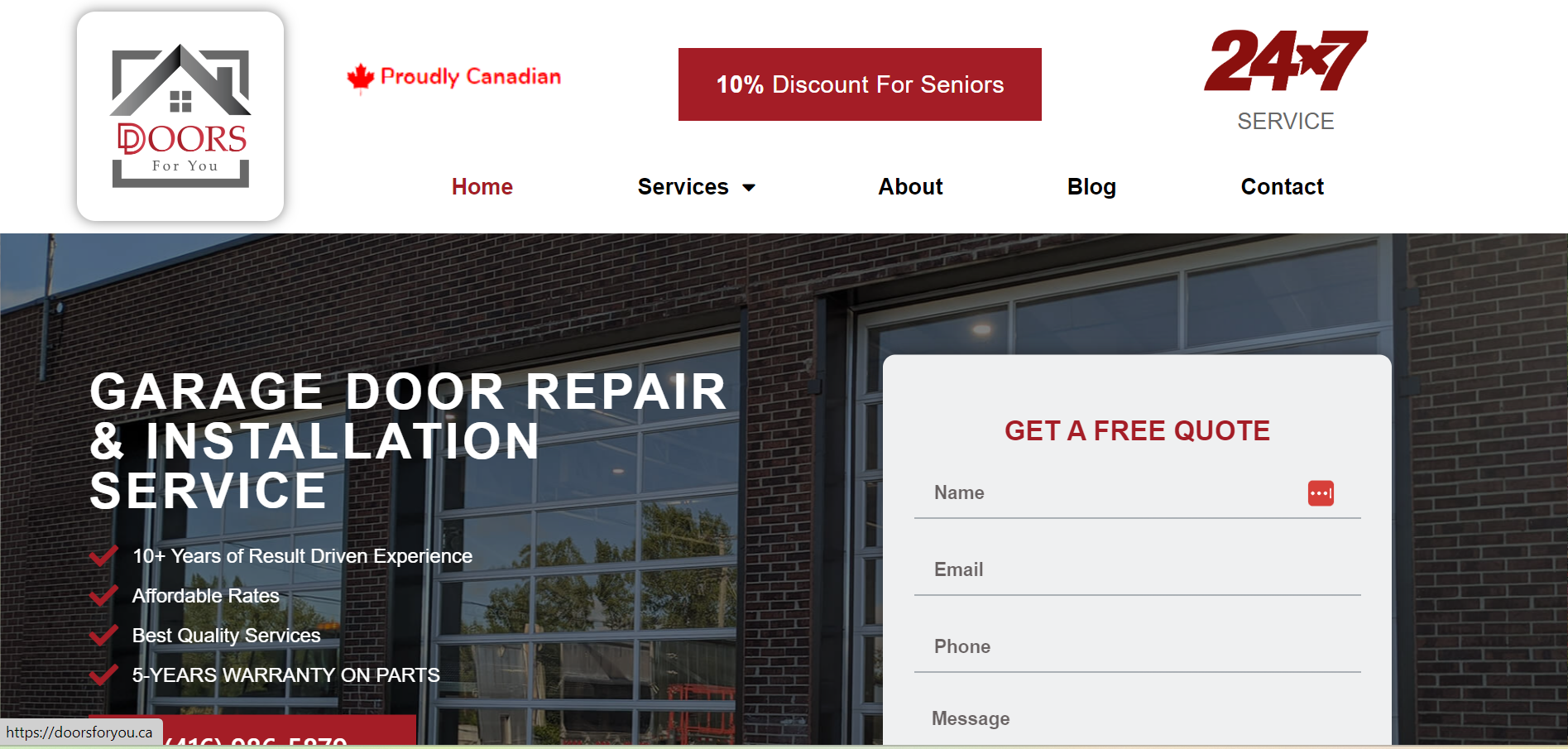A horizontally oriented screenshot of a comprehensive web page for a garage door repair and installation service. Dominating the center of the image is a central section showcasing essential service information, which includes a thin photograph of reflective garage windows, possibly representing a service station. The left side prominently features text that highlights key aspects of the service: "Garage Door Repair and Installation Service," "10 Years of Result-Driven Experience," "Affordable Rates," "Best Quality Services," and "5 Years Warranty on Parts."

On the right side, a conspicuous white pop-up box with red text invites visitors to "Get a Free Quote," accompanied by fields marked for Name, Email, Phone, and Message inputs. The web page is framed by a clean white strip serving as the top banner, which lacks a top border for a streamlined look. 

The upper left corner of the banner displays the "Doors For You" logo alongside the phrase "Proudly Canadian." Centrally positioned in the banner is a red button offering "10% Discounts for Seniors," and to its right, the assurance of "24 by 7 Service." 

Beneath the banner, five drop-down menu elements are presented: "Home" in red text, followed by "Services," "About," "Blog," and "Contact" in black text, providing clear navigation options. Additionally, at the lower left-hand corner of the screenshot, a small gray text box displays the web address: "https://doors4u.ca."